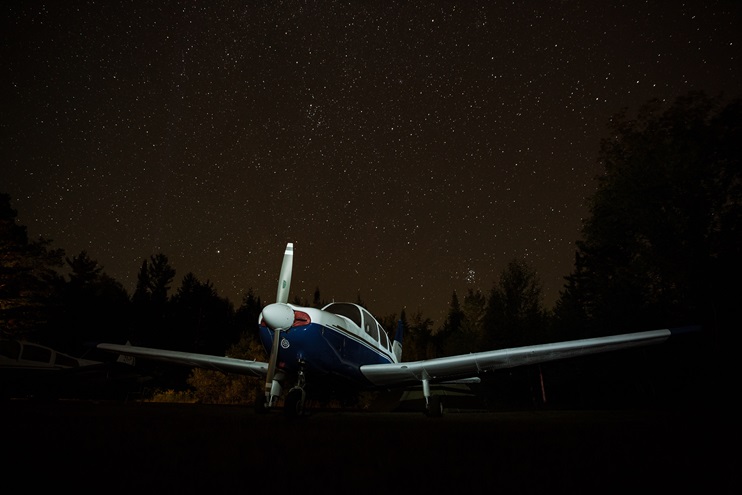A single-engine airplane is prominently displayed in a nighttime scene. The plane features a distinctive color scheme with a white nose, white propeller, and a white top with a blue bottom. Its white wings stand out against the night sky. The aircraft appears to be unoccupied, parked, and viewed from a slightly lower angle, revealing part of the wheel in shadow. The background is dark, suffused with a subtle brownish hue, and dotted with white stars. If you look closely, you'll discern the black silhouettes of trees and bushes against the dark backdrop. The lighting focuses primarily on the airplane, suggesting it might be a computer-generated image given the contrast with the surrounding darkness.